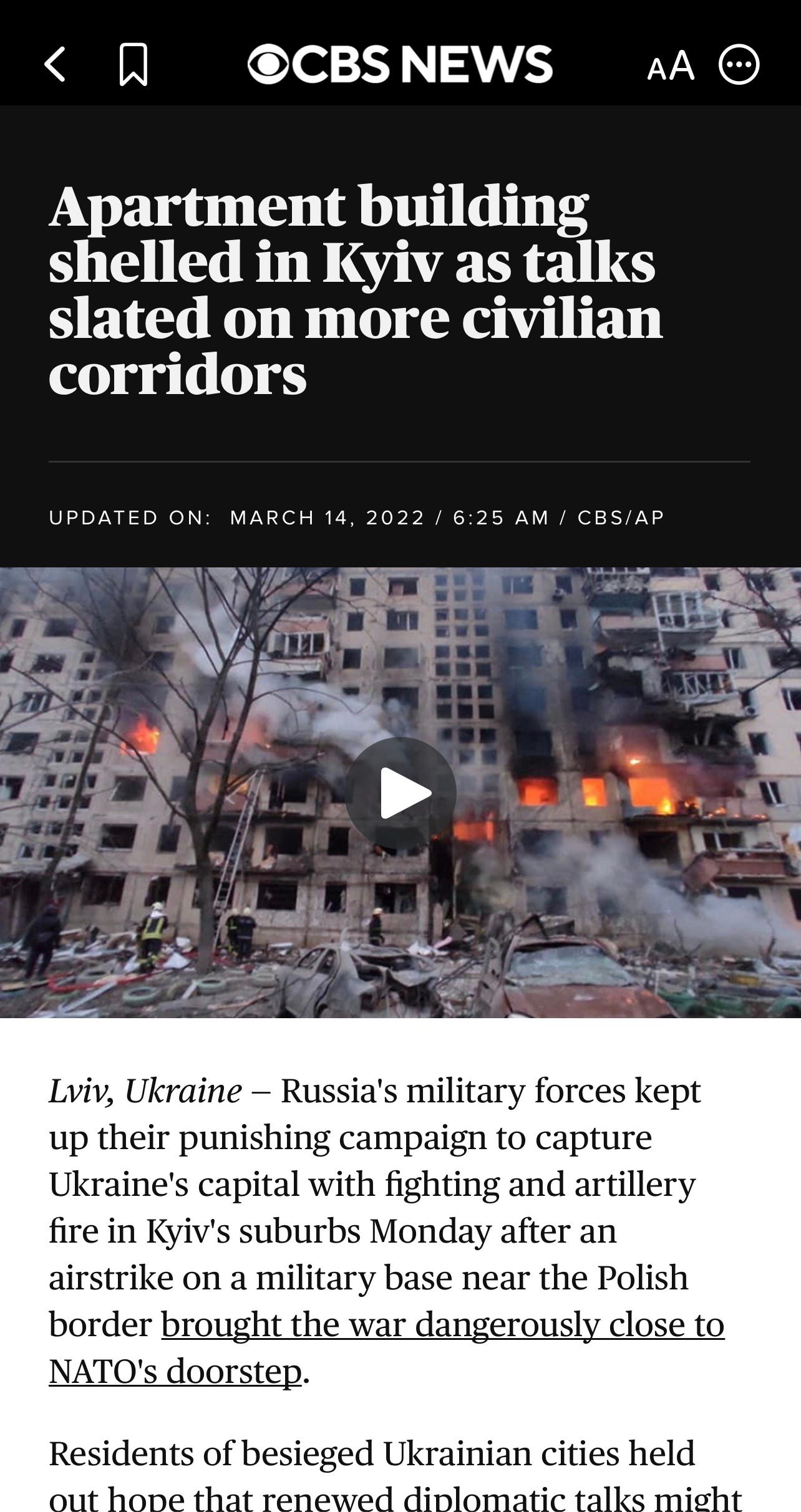In the upper half of the image, a news webpage presented in a dark theme prominently displays the banner "CPS News." Below this, the headline reads, "Apartment building shelled in Kiev as talks slated on more civilian corridors," with the update timestamp, "March 14, 2022, 6:25 AM CPS/AP." Centered beneath the headline is a video with a transparent black circular play button overlaid on the image.

The background scene of the video frame is a gray building engulfed in orange flames and grey, interspersed with dark smoke. In the foreground, a person wearing a navy jacket with green reflective strips stands to the left. Adjacent to a tree on the left side, a ladder leans against a window near the roof. Below the video, the text appears in black on a white background and reads: 

"Lviv, Ukraine — Russian military forces kept up their punishing campaign to capture Ukraine's capital with fighting and artillery fire in Kiev's suburbs Monday, following a strike on a military base near the Polish border, which brought the war dangerously close to NATO's doorstep. Residents of besieged Ukrainian cities held out hope that renewed diplomatic talks might end the conflict."